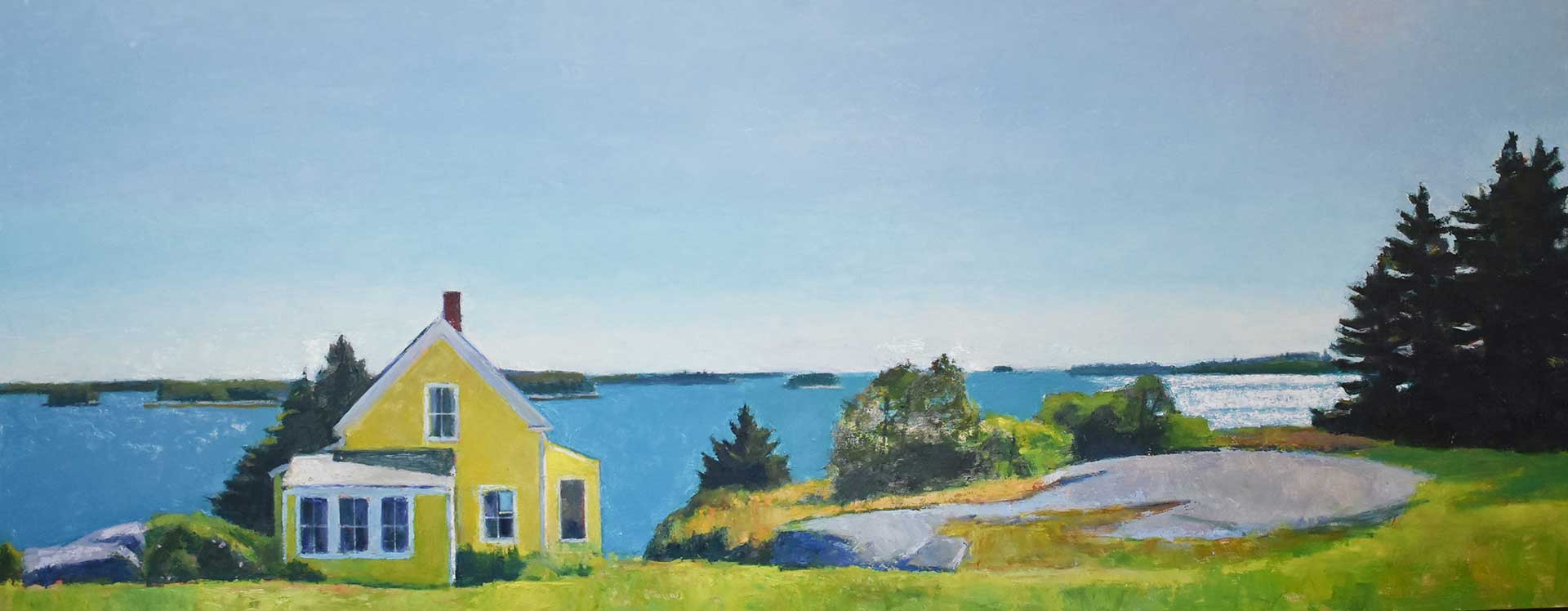This idyllic and peaceful painting captures a beautiful outdoor panoramic scene during daytime. Dominating the left side of the rectangular composition is an adorable, country-style yellow home. This two-story cottage features a quaint enclosed sun porch with three windows, a front door, and an additional window upstairs. The roof is white, and a single chimney stands out. Surrounding the house, the lush green grass suggests a warmer climate or season.

In the background, a serene body of water stretches out, dotted with small, grassy islands or atolls. Both left and right of the home are framed by trees, particularly pine trees on the right. A distinctive flat rock outcropping further enhances the natural charm of the scene. The blue sky above is lightly adorned with soft, shadowy clouds, and you can see where the sky meets the ocean on the horizon. The entire composition exudes a sense of tranquility and picturesque beauty.